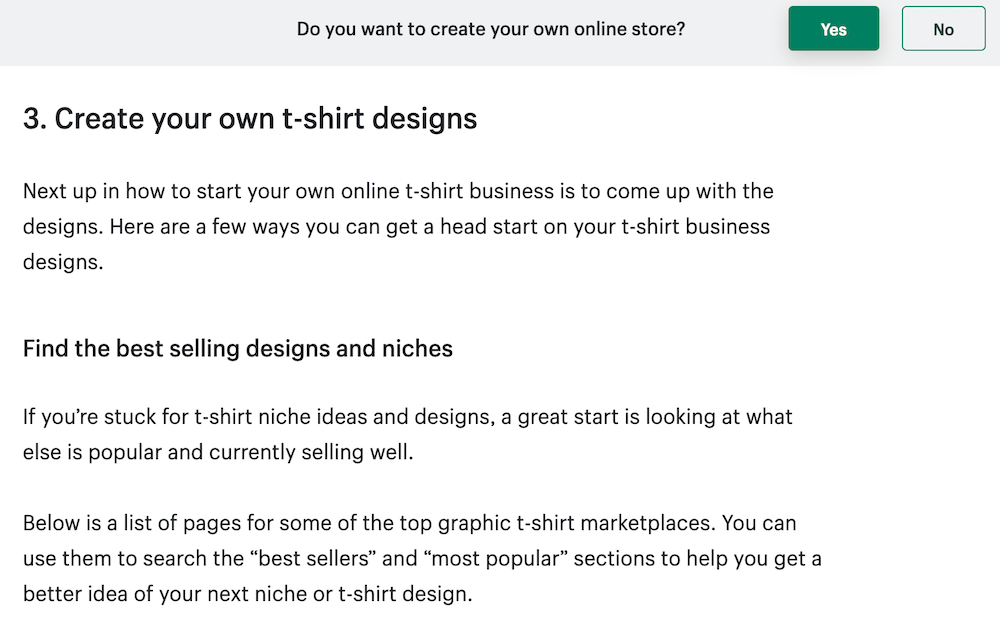The image represents a section of a website that offers guidance on starting your own online store, specifically focusing on creating and selling t-shirts. The top of the webpage features a gray border with the question "Do you want to create your own online store?" accompanied by two clickable buttons: a green "Yes" button on the left and a white "No" button on the right.

Below this header, a numbered step is indicated with a prominent "3" next to the text "Create your own t-shirt designs." A brief description follows, stating: "Next up in how to start your own online t-shirt business is to come up with the designs. Here are a few ways you can get a head start on your t-shirt business designs."

The content then shares a useful tip: "Find the best selling designs and niches. If you're stuck for t-shirt niche ideas and designs, a great start is looking at what else is popular and currently selling well." Furthermore, it mentions a list of pages from top graphic t-shirt marketplaces to help users search the best-selling and most popular sections for inspiration on their next t-shirt niche or design.

The background color of this section is white, and the text is in black, ensuring clarity and readability. There is a noticeable gap between the number "3" and the subsequent text "Create your own t-shirt designs," providing a clean and organized layout.